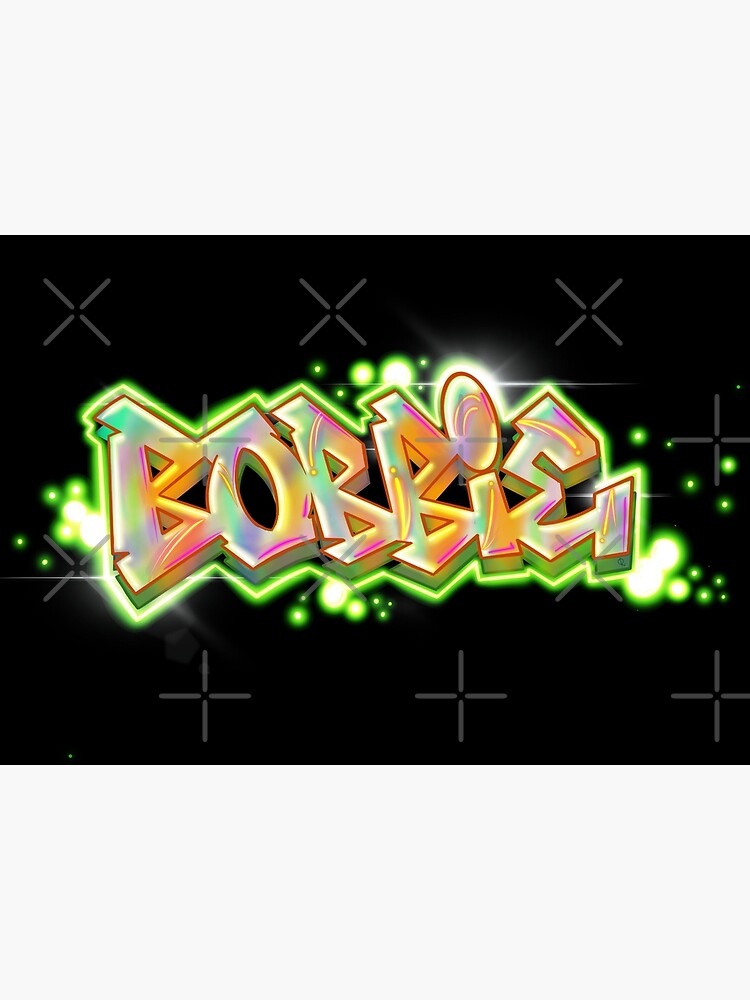The image features a vibrant piece of street art that depicts the word "Bobby," spelled out as B-O-B-B-I-E, in bold, block letters. The letters are adorned with a gradient of striking colors such as gold, silver, rose, orange, and yellow, and are outlined in bright neon green with hints of white, giving the impression of being illuminated. The dot over the "I" is accented with a painted lens flare, adding a touch of realism to the graffiti. The background is solid black, featuring various X's and crosses in a lighter shade of black, scattered across the image. Additionally, small green dots are artistically placed around the letters. This combination of elements evokes the distinct style of street graffiti typically seen on buildings and train cars. The meticulous detail and blend of colors suggest that this artwork might be available as purchasable clip art.